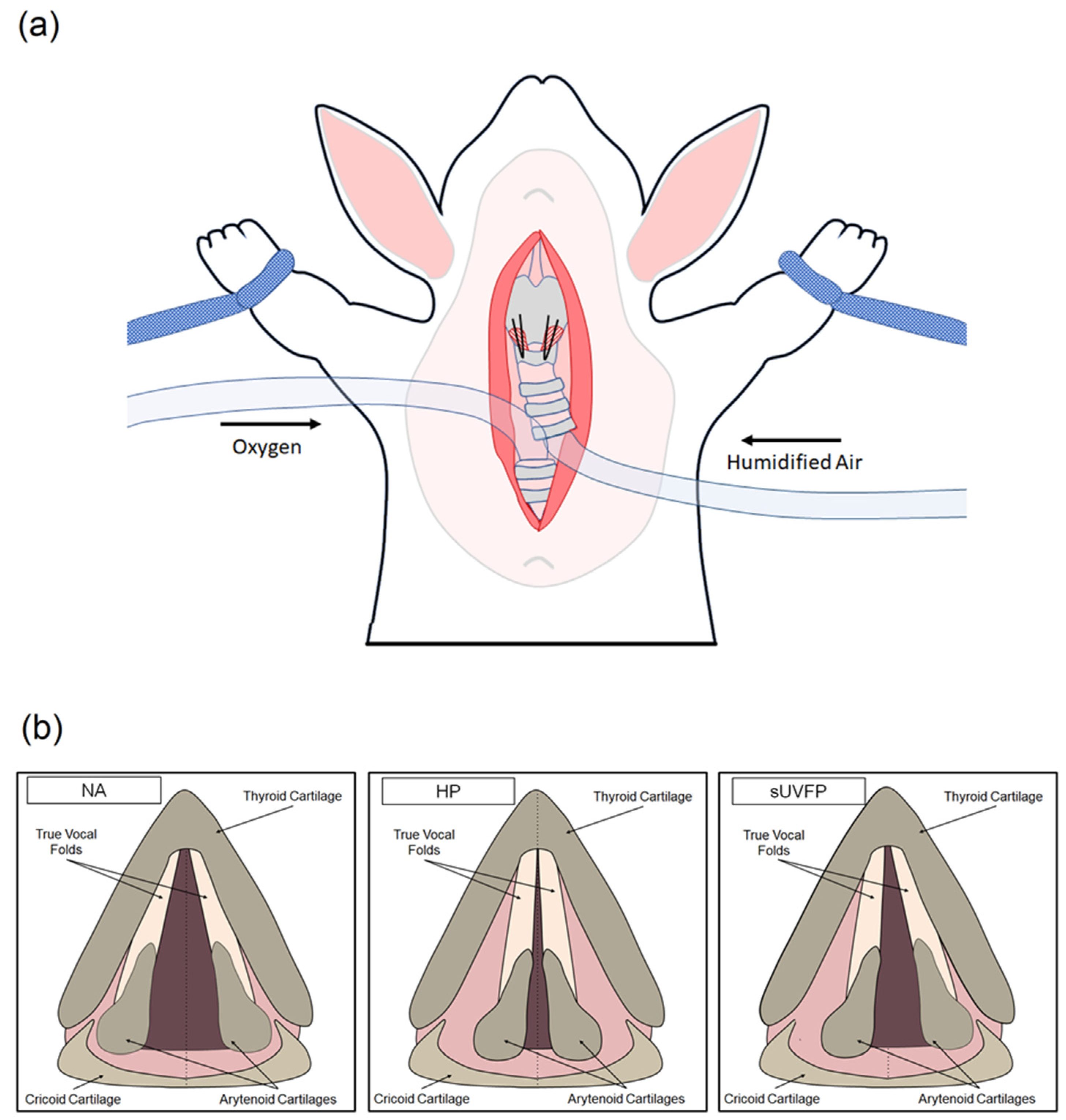The image is a detailed medical illustration, primarily depicting an animal, possibly a rat, in a subdued state, lying prone with its wrists tied with blue lines. The main diagram, labeled as Diagram A, showcases the animal's windpipe with oxygen being delivered via an arrow pointing to the right and humidified air being expelled via an arrow pointing to the left side of the animal. Below this, Diagram B comprises three square panels, each focusing on different anatomical features of the throat. The leftmost panel (labeled "NA") highlights the thyroid cartilage, true vocal folds, cricoid cartilage, and arytenoid cartilage. The middle panel (labeled "HP") illustrates the same parts in more detail. The right panel (labeled "SUVFP") continues to emphasize the true vocal folds along with other cartilage structures. This comprehensive depiction provides specific insights into the workings and structure of the animal's respiratory and vocal anatomy.